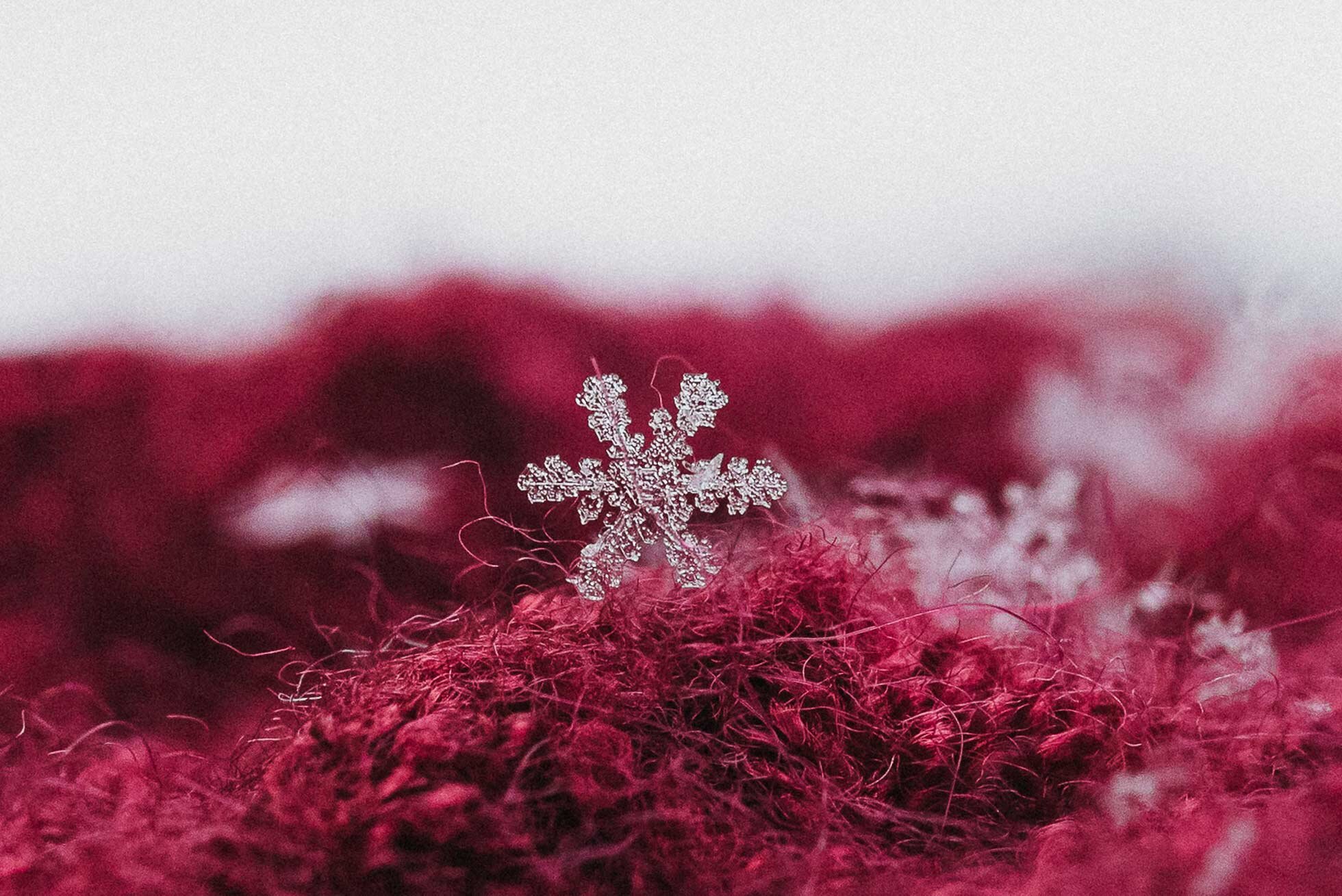This detailed macro photograph features a centrally positioned, plastic, six-sided snowflake decoration, possibly intended for use as a Christmas tree ornament or even a necklace. The snowflake, starkly white with slight off-grey hues, stands vertically amidst a vibrant, deep wine red background. The red material underneath, which could be a jumper, carpet, jacket, rug, or sweater, is heavily textured with fibrous threads closely resembling a bird's nest or bundled shrubbery. The blurred background continues in the same vivid red, accentuated by sporadic patches of white fibers, contributing to its intricate and striking composition. The overall scene lacks any identifying details such as names, text, or location, allowing the intricate artistry of the snowflake and the red fibrous backdrop to remain the focal points.